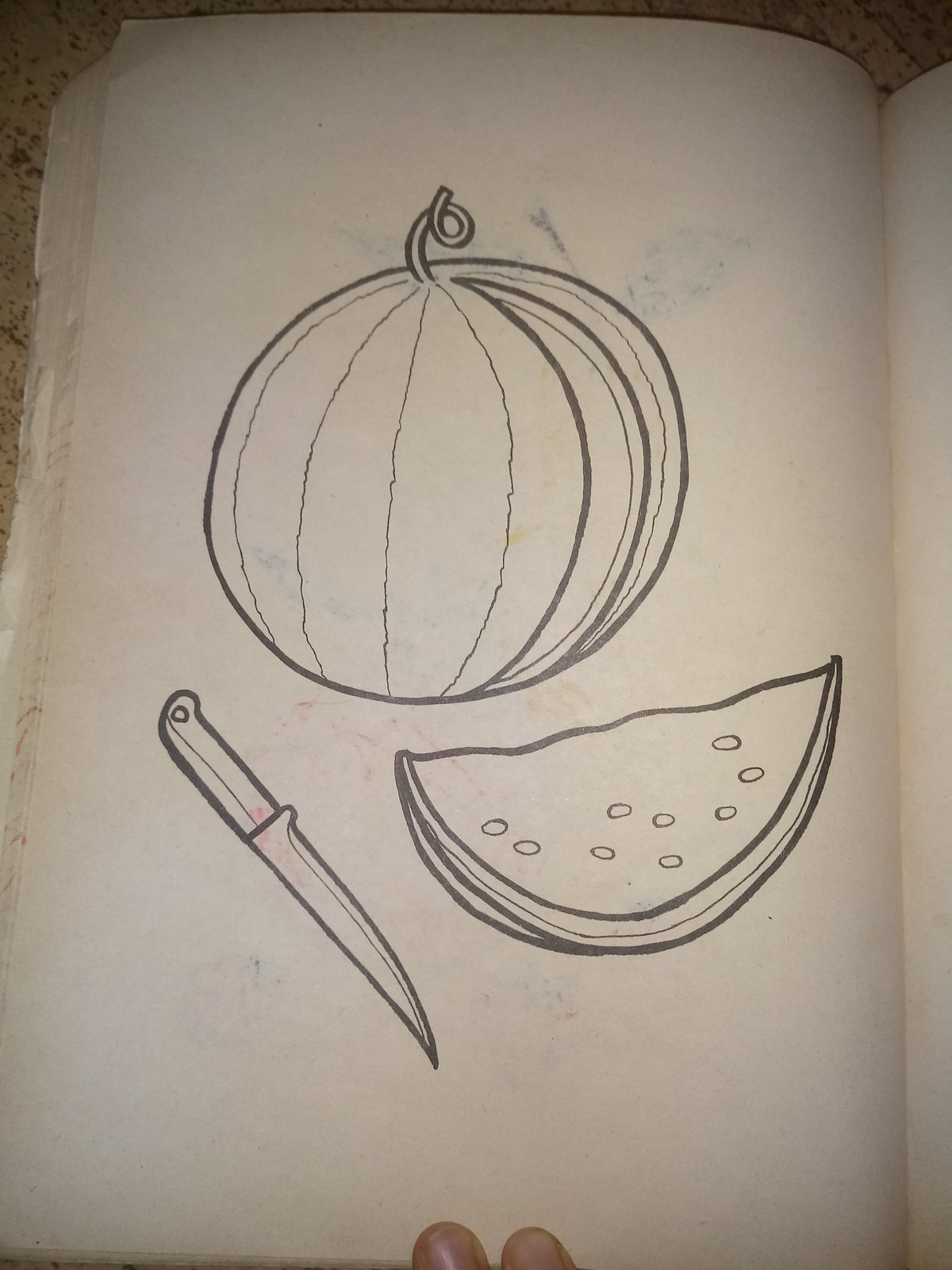This indoor photograph captures a page from a slightly browned sketchbook viewed from above. Dominating the composition is a detailed line drawing of a round melon near the center, depicted with vertical segments and a curly, pigtail-like stem. The melon is missing a wedge on the lower right side. To the left of the melon, a paring knife is illustrated with its handle directed towards the upper left and its blade pointing to the lower right, aimed towards the center bottom. Right of the melon, the removed wedge is shown laid on its side with about ten simple oval shapes representing the seeds. Towards the bottom edge of the photograph, two visible fingers are holding the page down, revealing that it is part of a sketch pad. The adjacent pages show faint bleed-through of other drawings. The illustration is executed with black marker or pen, and there are no words or text present in the image.